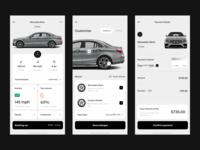This detailed caption summarizes an image comprising three mobile app interface screens designed for a car rental or purchase service, specifically for a Mercedes-Benz vehicle. The app's interface is sleek, modern, and user-friendly, predominantly featuring a monochromatic silver color scheme.

The first screen provides comprehensive vehicle details at the top, showcasing an image of a Mercedes-Benz car. Below the image, specific details such as top speed (101 miles per hour) and mileage range (256 miles) are provided. Additionally, two gauges display extra information: a speedometer at 141 miles per hour and a battery indicator at 68%. Towards the bottom, a "Book Now" button is available, accompanied by the price of $215 and an "Add to Cart" option.

The second screen focuses on vehicle customization. It features a rear view of the Mercedes-Benz car at the top and prominently displays a "Customize" button. Two customization options are listed—Mercedes-Benz rims and custom black rims—each with a selection button. A "Save Changes" button is situated at the bottom of the screen.

The third screen displays payment details. An image of the front of the Mercedes-Benz car is shown at the top, alongside detailed payment information, including monthly installments of $750 for the Mercedes-Benz. A "Confirm Payment" button is positioned at the bottom of the screen.

The overall design emphasizes clarity, ease of use, and a streamlined process for viewing, customizing, and purchasing or renting a vehicle. However, the simplicity and user-friendliness of the app design may evoke concerns about its legitimacy.